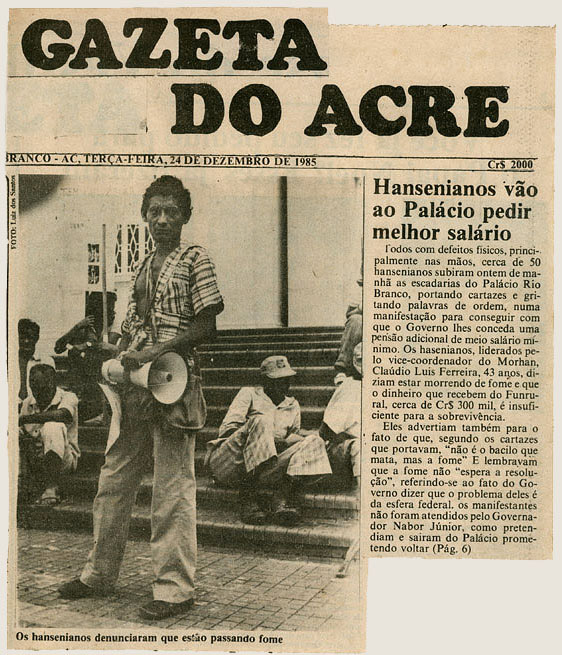The image centers on an old newspaper article titled "Gazeta de Uyghur," dated December 1985, written predominantly in Spanish. The article is positioned against a white backdrop, prominently displaying black, gray, tan, and white hues. The main focus of the article is a black-and-white photograph located in the bottom left corner. The photograph features a man standing in front of a staircase, holding a loud megaphone in his left hand and facing forward, wearing a multicolored shirt and pants. Flanking this man are several people, some seated on the steps to his left and right, with varied postures and gazes. The article itself runs down the right-hand side of the newspaper, consisting of three headline lines followed by two paragraphs. The text mentions "D.O. A.C.R.E." under the main title, though part of it appears obscured or cut off. The setting is outdoors, likely taken in the middle of the day, capturing a moment in what appears to be a significant event or gathering.